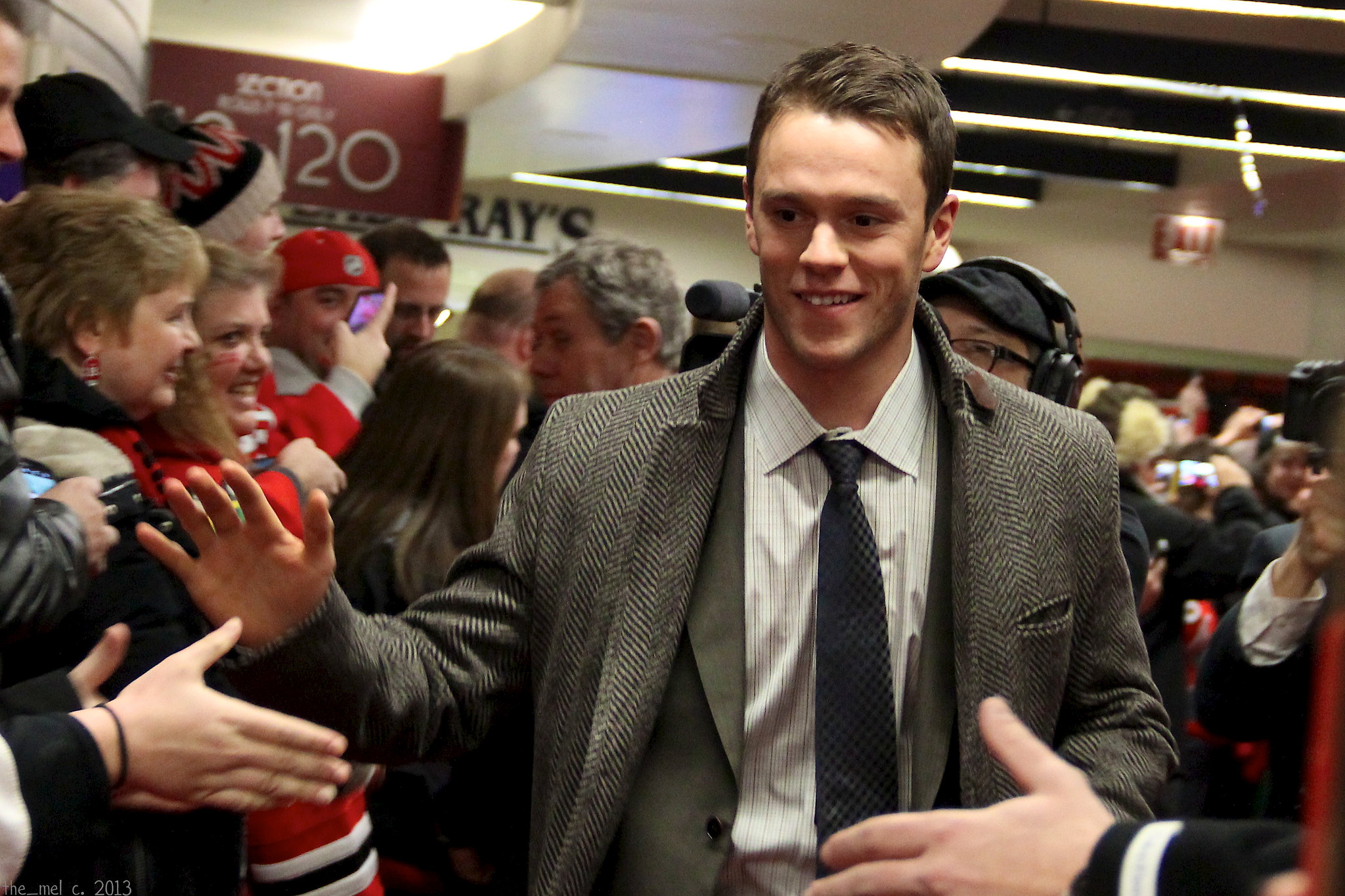In the photograph, a man in his 20s or 30s, with black hair, is seen walking through a crowd, only visible from his waist upwards. He is dressed in a black and white twill jacket with a front coat pocket on the chest, under which he wears a dark green business coat paired with a white and gray striped button-up shirt and a black and gray striped necktie. The man is smiling warmly and looking towards someone in the bottom left corner of the frame, while waving his hand or making a motion as if to clasp or shake hands with someone. The crowd around him is joyful, with people smiling, clapping, and focusing their attention on him. Positioned behind the man, a person is visible holding a camera and wearing headphones, adding to the lively and engaging atmosphere of the scene.